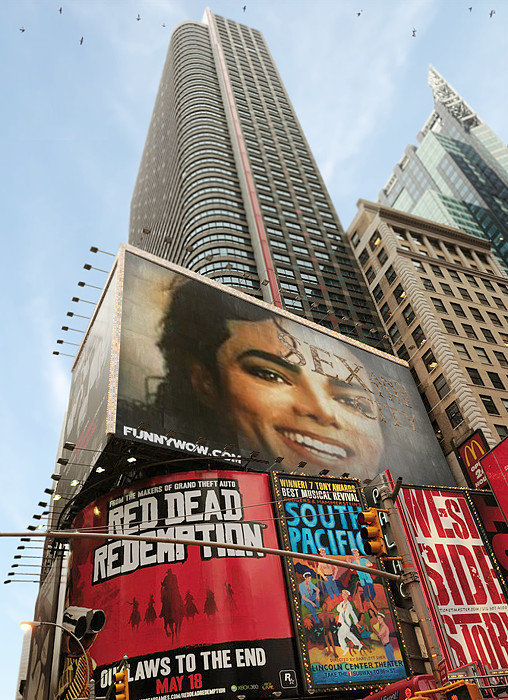The color photograph captures the bustling atmosphere around Times Square in New York City, showcasing an iconic array of vibrant, large billboards at the base of towering skyscrapers. The perspective of the image is angled upwards at approximately 45 degrees, providing a dynamic view that stretches from the bustling streets to the sky. Among the billboards, there is a prominent one featuring a picture of Michael Jackson, another advertising "West Side Story" with bold red lettering on a white background, and a bright blue "South Pacific" billboard depicting people dancing on a beach. Additionally, a striking image for "Red Dead Redemption: Outlaws to the End" shows cowboys riding in a scene with white and black text against a red backdrop. The scene is detailed further with overhead lights protruding from the top of the billboards, intended to illuminate them at night. In the bottom left and top right corners of the photograph, yellow traffic lights positioned on utility poles confirm the unmistakable backdrop of New York City. The clear daytime sky, with wisps of white clouds and birds flying just above the height of the skyscrapers, adds to the overall sense of depth and liveliness in this quintessential urban setting.